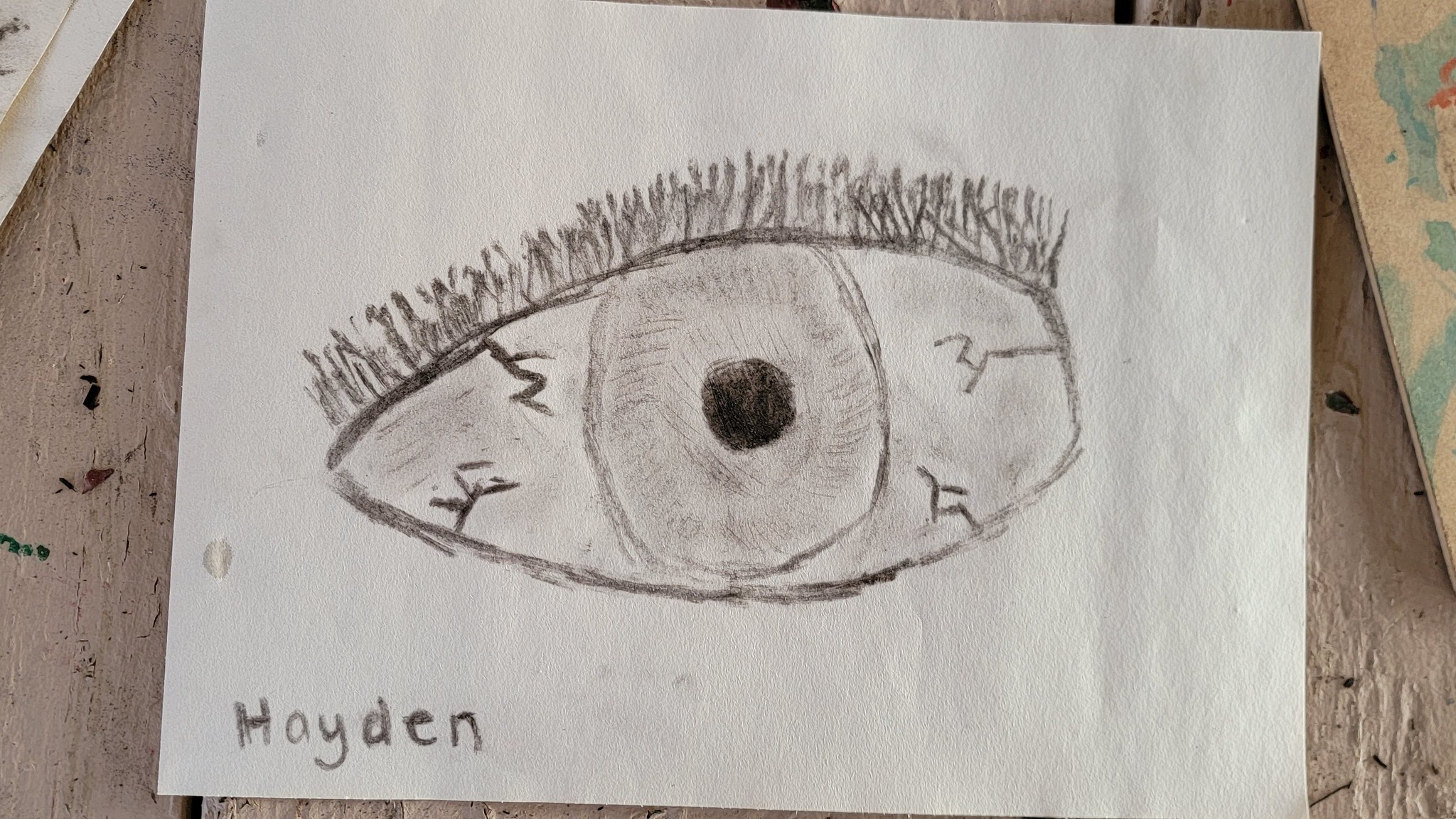This image features a detailed black-and-white sketch of an eye on an off-white sheet of paper. The eye is framed with meticulously drawn eyelashes extending from the top. The contours of the eye form a teardrop shape, oriented towards the left edge of the page. At its center, the eye has a large, lightly shaded pupil with a stark black circular core. Fine lines depicting veins radiate within the eye, adding a sense of realism. Along the bottom left corner of the sketch, the name "Hayden" is printed in bold black letters, likely indicating the artist's name. The paper rests on a light taupe-colored wood surface, with indistinct objects cropped out on the left and right sides of the image—suggesting a brown item on the right and a white paper-like object on the left.